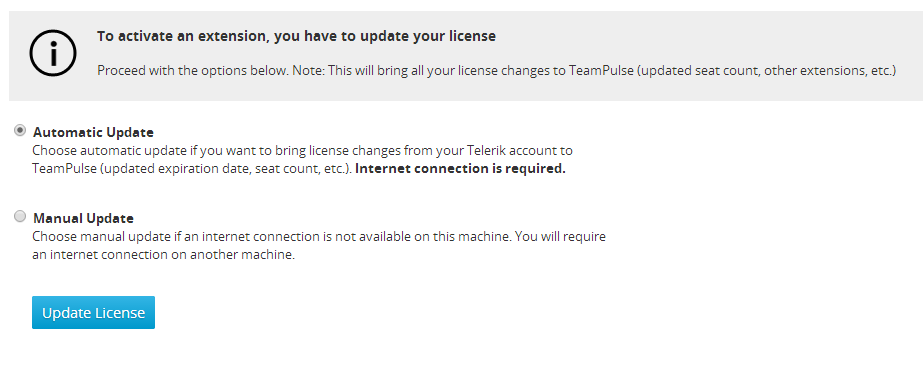The image features a structured user interface for updating a software license. 

At the top of the image is a light gray banner. In the upper left corner of this banner, there is a black circle with the letter "I" in the center, also in black. Adjacent to this, a dark black text runs across the top, reading, "To activate an extension you have to update your license." Below this, in medium gray text, it says, "Proceed with the options below. Note, this will bring all your license changes to Team Pulse, updated seat count, other extensions, etc."

The main part of the page has a white background featuring two update options, each accompanied by a selection circle. 

1. **Automatic Update**: 
   - The selection circle next to this option is filled with a black dot.
   - In dark text, it says, "Automatic Update."
   - Below this, in lighter gray text, "Choose automatic update if you want to bring license changes from your Telerik account to Team Pulse. Updated expiration date, seat count, etc."
   - In darker text, it underscores, "Internet connection is required."

2. **Manual Update**:
   - The selection circle next to this option is not filled.
   - In black text, it says, "Manual Update."
   - Below, in lighter gray text, it reads, "Choose manual update if an internet connection is not available on this machine. You will require an internet connection on another machine."

At the bottom of the page, there is a rectangular button with a blue background, featuring the text, "Update License," in white.